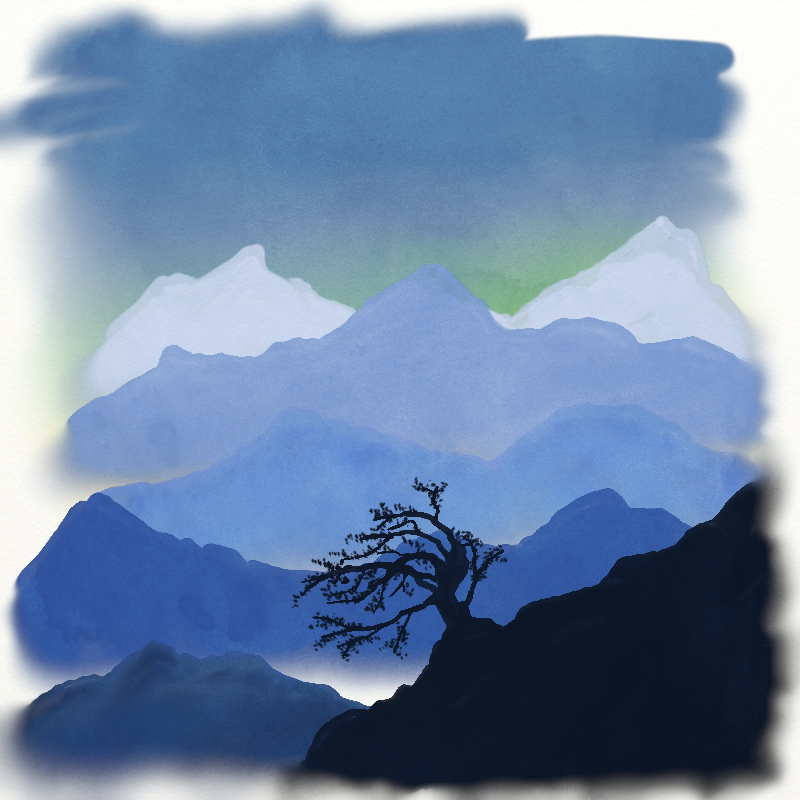This square painting showcases a minimalist yet evocative scene using a limited palette of colors: black, dark blue, medium blue, light blue, sky blue, light gray, light green, and periwinkle dark blue. The edges of the sky appear to have been spray-painted, with white specks creating a textured, almost ethereal effect that suggests the use of a stencil. Dominating the foreground is the stark black silhouette of a short and stubby tree with wide, gnarly branches stretching in various directions — some pointing up, others down, and several arching over. The landscape begins at the bottom right, extending into the scene as another black silhouette. Beyond this, a series of mountains recede into the distance, depicted in a gradient of blue hues that enhance the sense of depth. The furthest mountains are capped with snow, rendered in a light gray that contrasts with the light green and periwinkle blue sky above. The careful arrangement of colors and shapes not only conveys a tranquil landscape but also evokes a sense of quiet majesty in nature's simplicity.